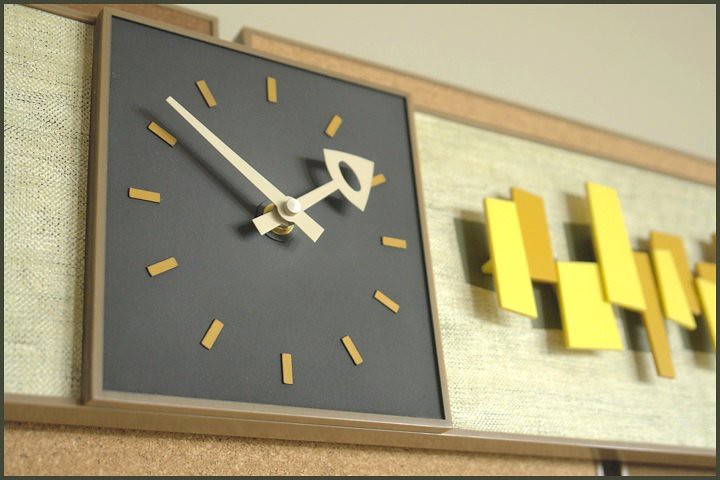The image centers on a square clock, which stands out against a sleek black backdrop marked with minimalist gold slashes to indicate the hours. The clock features a bold white hour hand, distinguished with a unique triangular tip containing an oval opening, and a matching white minute hand. The clock is mounted on a larger rectangular canvas-colored surface, which serves as a subtle, elegant backdrop. Surrounding the clock is a cluster of neatly arranged rectangular yellow shapes, adding a dynamic and modern artistic element to the overall design.